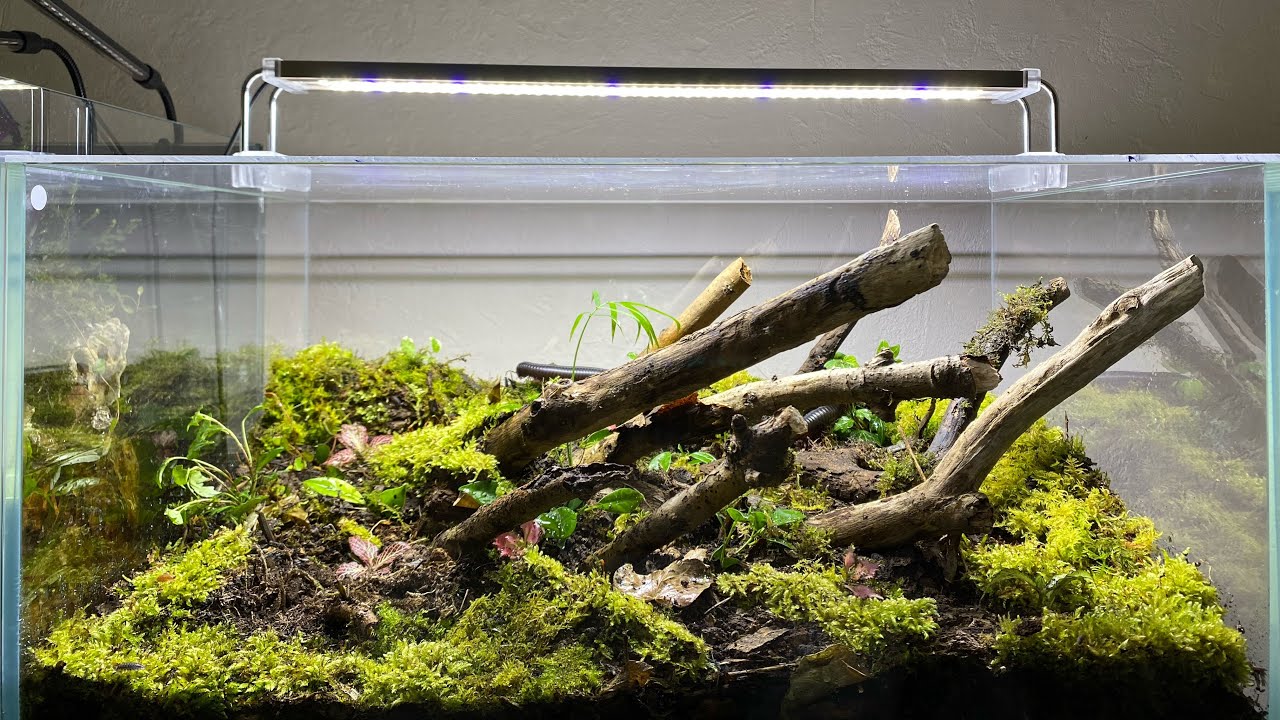The image displays a rectangular terrarium made from clear acrylic or glass, resembling a fish tank. It features a silver, long, flat handle across the top for lifting the cover. Set against an off-white wall, the interior base of the terrarium is covered with dirt. Scattered throughout are pieces of driftwood, resembling thin tree trunks, oriented almost horizontally. The bottom is carpeted with moss, surrounding vibrant greenery that includes light green grasses and a sturdy, taller plant with narrow leaves similar to a palm tree. The driftwood branches reflect against the terrarium's walls, creating a sense of depth. Although the terrarium environment includes soil, moss, and various plants, no visible animals appear within, suggesting any inhabitants might be well camouflaged. A lamp shines from above, likely serving to provide warmth, essential for any cold-blooded creatures that might reside inside.